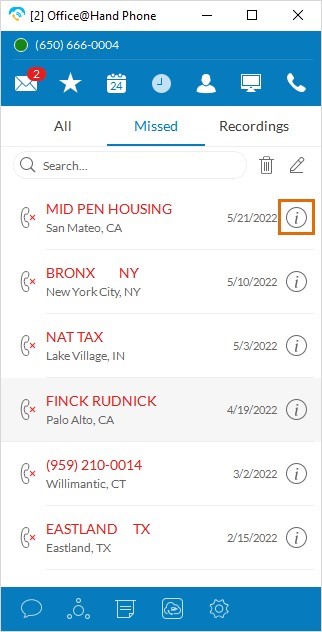The image showcases a mobile app interface, presumably for managing office communications. At the top left corner, the header reads "Office at Handphone," preceded by a yellow telephone icon and followed by the number "2" in brackets. On the top right are three standard window control icons: an "X" for closing, a square for maximizing, and a minus sign for minimizing.

Below this header, a green circle displays the contact number "650-666-0004." Further down, seven distinct icons are aligned horizontally, representing different features: an envelope for messages, a star for favorites, a calendar with the number "24" for events, a clock for recent activities, a profile icon for contacts, a monitor for screen sharing or display, and a telephone for call history.

In the center section, three tabs labeled "All," "Missed," and "Recording" are visible, with "Missed" highlighted in blue, indicating it is currently selected. This tab displays six missed calls, each highlighted in red for emphasis. Additionally, the first missed call entry is marked with an orange square enclosing a circle with an 'i,' likely indicating important information or a detail alert for that call.